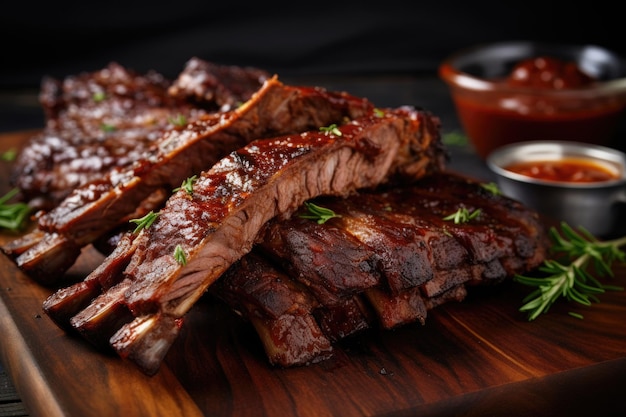This is a detailed close-up photograph of a mouth-watering barbecue rib dish, brilliantly staged for visual appeal. The ribs, which could be either beef or pork, are generously coated in glossy barbecue sauce, making them glisten under the light. Arranged meticulously on a dark wooden slab or butcher block, the presentation features multiple racks of ribs layered horizontally at the base, with additional sliced ribs artfully draped over the top. Sprinkled with pieces of fresh rosemary, the ribs are garnished with a full sprig for added aromatic flavor. In the background, there are two containers of sauces: a clear glass bowl, presumably filled with barbecue sauce, and a smaller metal ramekin, possibly containing salsa or additional barbecue sauce. The entire setup evokes the kind of hearty, well-crafted meal you might expect to find in a high-quality restaurant.